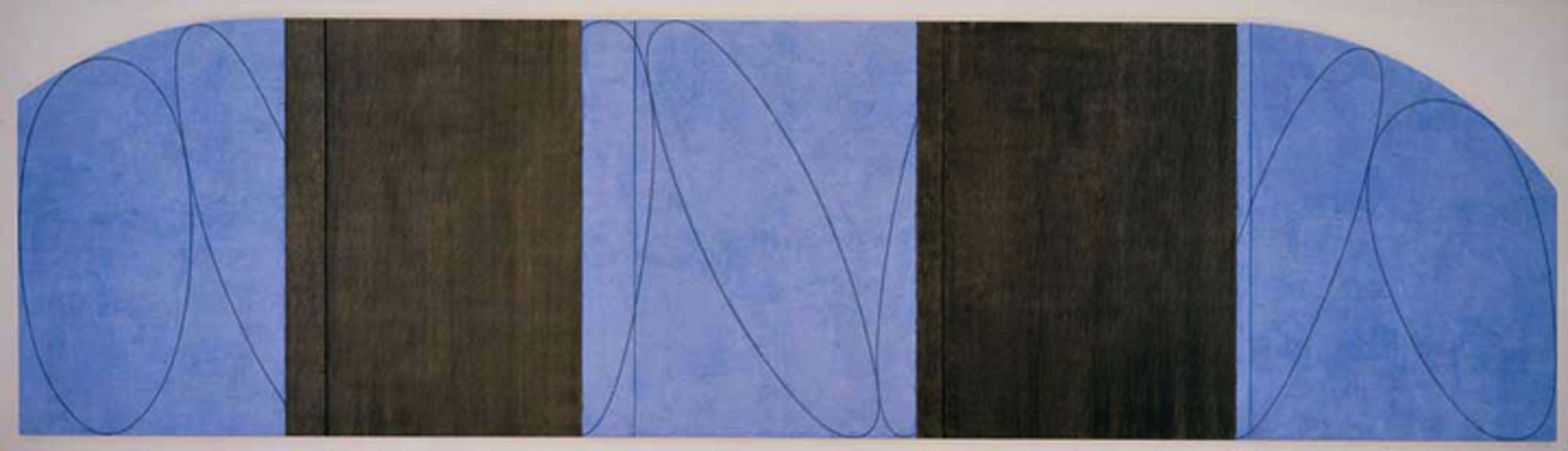The image is an abstract artwork with a primarily horizontal composition. It features a rectangular shape with both the top left and right corners curved inward, deviating from a perfect rectangle. The artwork is divided into five alternating sections: three blue and two gray. The gray serves as a background and a border around the image, while the blue panels contain a series of darker blue ovals, which lean in varying directions—some overlap and extend from right to left, while others go left to right. Notably, the central blue panel is slightly lighter than the other blue sections. The pattern alternates between blue sections with ovals and plain black stripes. The overall appearance is that of an intricately designed pattern comprising contrasting blue and black stripes, with detailed oval motifs in each blue section.